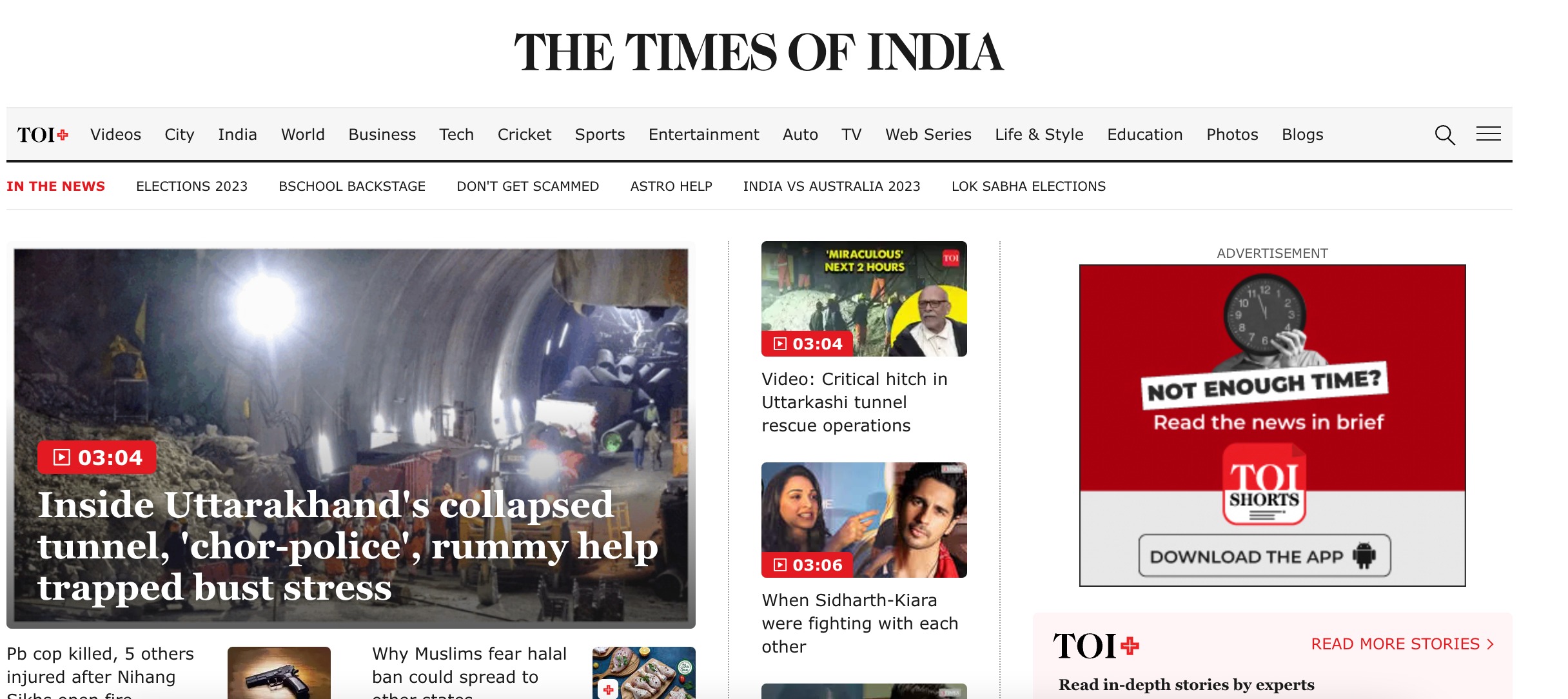Caption: 

A detailed screenshot from "The Times of India" news website showcases its homepage, currently centered around major current events. The website’s title, "The Times of India," is prominently displayed in a large, bold, capitalized Serif font, center-justified, with the iconic TOI logo and a red diamond positioned to the left. The main navigation menu horizontally spans the top of the page, offering a variety of sections: Video, City, India, World, Business, Tech, Cricket, Sports, Entertainment, Auto, TV, Web Series, Life & Style, Education, Photos & Blogs. It includes a search icon represented by a magnifying glass and a hamburger menu.

A 3-pixel grey line divides the main header from the content. Below, in bold text on the left, is the "In the News" section featuring various topics like Elections 2023, B-School Backstage, Don't Get Scammed, Astro Help, Ind vs. Australia 2023, and Lok Sabha Elections, with each title in capitalized regular text.

On the left side of the screen, a large image highlights a news video titled "Inside Udara Khan's Collapsed Tunnel," captioned with the phrase "Chor-Police, Rummy Help Trap to Bust Stress." The image reveals people and construction materials inside a tunnel illuminated by large lights. Below this primary feature are smaller thumbnails linking to additional stories.

The center column features more video content, including "Critical Hitch" and "Udakari's Tunnel Rescue Operations," with corresponding thumbnails. Another video titled "When Sid, Hartha, Kiara were fighting with each other" shows a woman pointing at a man in its thumbnail. The topmost video depicts a person on top of a tunnel, adding to the visual narrative of the ongoing crisis.

On the right side, a prominent ad encourages readers to "Read the news in brief" by downloading the TOI app, promoting access to "Top Stories by Experts." This visual invitation underscores the convenience of staying informed through mobile access.